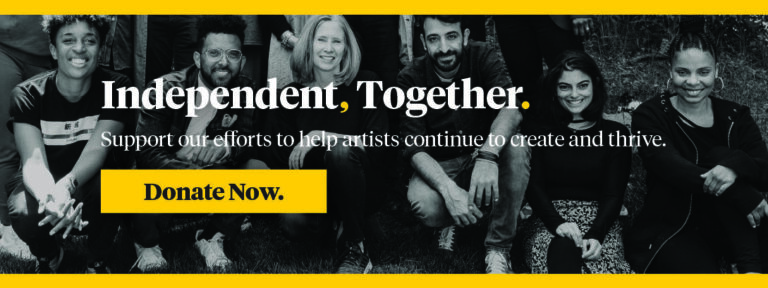A rectangular section of a web page features a black-and-white image with thin yellow borders at the top and bottom. The image captures six individuals seated or squatting in a row, posed outdoors on a grassy area. From left to right, the visible individuals include a Black male, a male possibly of Middle Eastern descent, a Caucasian female, another male, an ambiguous female, and a Black female. In the background, partially cut off, are five more people standing.

The image is overlaid with white text that reads, "Independent, Together." Independent is followed by a yellow comma and together by a yellow period. Below, it states, "Support our efforts to help artists continue to create and thrive." At the bottom, within a yellow box and in black text, it says, "Donate Now."